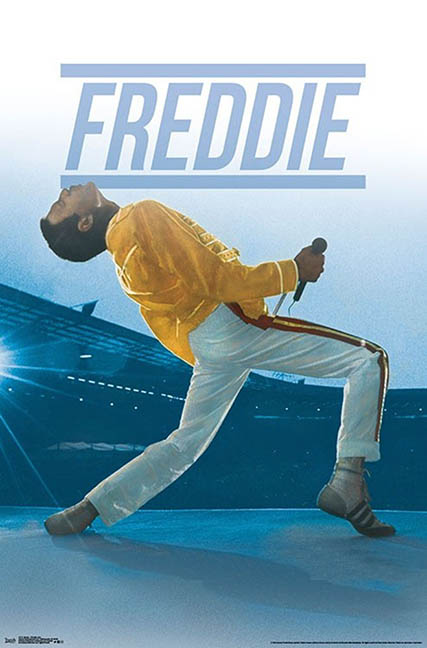This vibrant color photograph captures the iconic Freddie Mercury, the legendary lead singer of Queen, during a powerful live performance likely from the 1970s or 1980s. Freddie, dressed in a striking yellow silk shirt and white pants accented with a bold red and yellow racing stripe, exudes energy and charisma. His high-top tennis shoes add to his dynamic stage presence. In the image, Freddie is leaning back with his head, mouth, and chin pointed skyward, as if he's singing with immense passion. He clutches a microphone in his hand, captivating the audience in an outdoor arena at what appears to be dusk or twilight. A dramatic stage light shines from the mid-left of the frame, adding to the electrifying atmosphere. The retro vibe of the photograph is amplified by the bold blue text at the top that reads "FREDDIE," framed by horizontal lines above and below, underscoring the larger-than-life presence of this legendary performer.